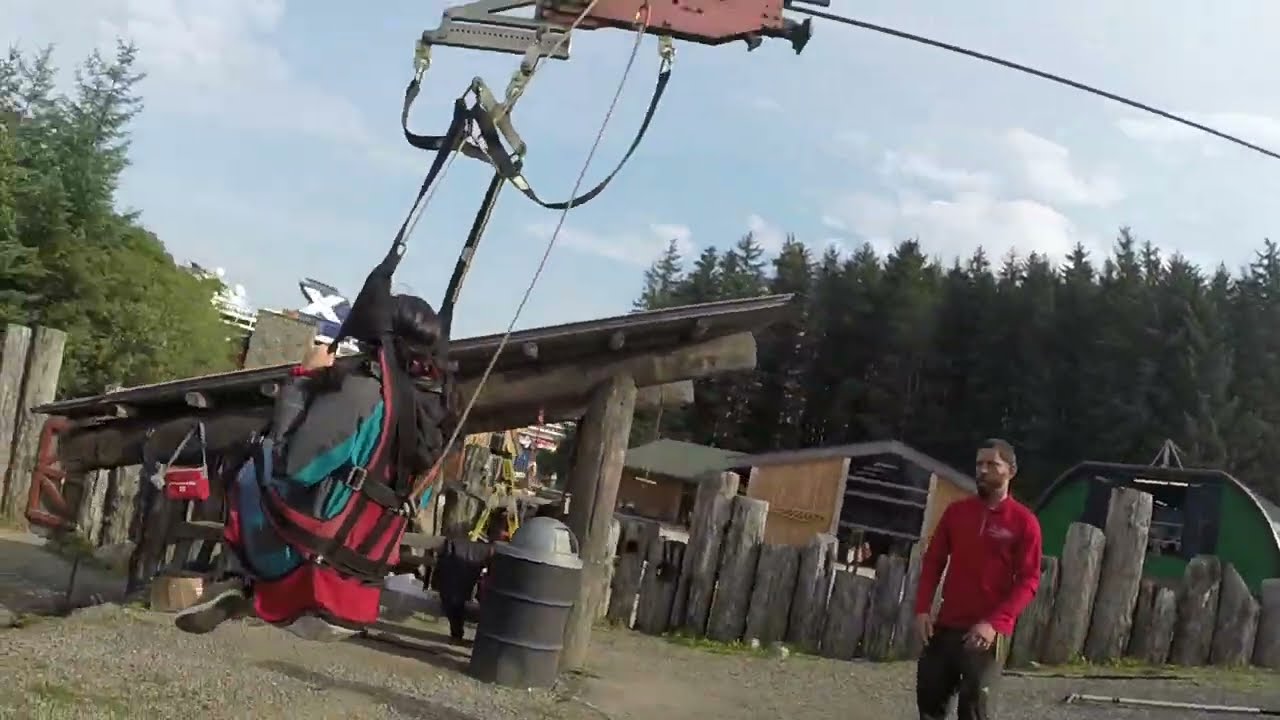The image captures a picturesque outdoor park setting featuring a zipline setup. In the foreground, a woman is seated in a red sling chair harness, which is sturdily attached to a winch system by black straps. She appears to be near the end of the zipline ride, gripping the sides of the harness with her feet scrunched up beneath her. Approximately ten feet in front of her stands a short-haired man with a beard, dressed in a red shirt with a company logo and dark pants, likely an employee ready to assist her. Adjacent to the man is a solar-panel-topped structure, possibly a seating area with a trash can nearby.

The mid-ground is dominated by a rustic fence composed of large, uneven timber logs, adding to the park's natural aesthetic. Behind the fence is a small building hinting at a recreational center, framed by pine trees on its right side. The entire scene is enveloped in a serene, forested environment, offering a blend of adventure and tranquility.